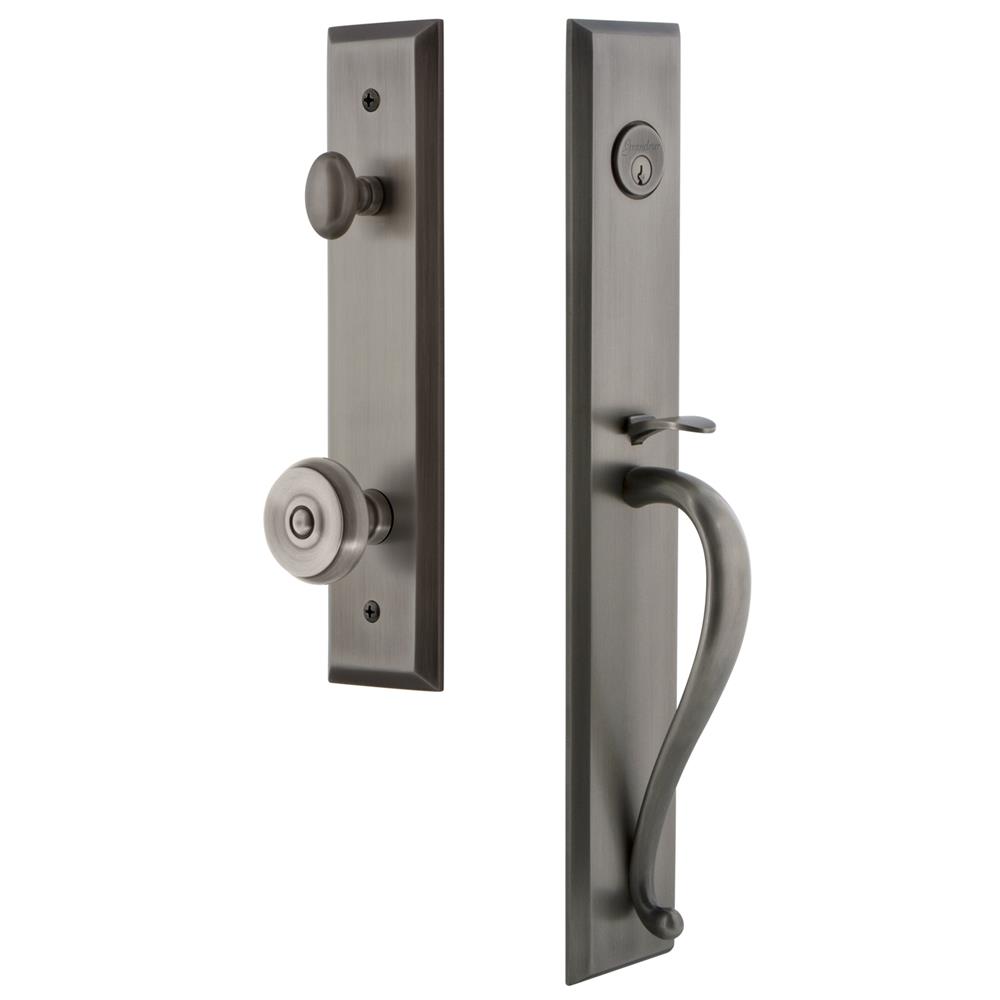This image showcases two types of door locking mechanisms mounted on separate rectangular metal plates. The plate on the left features a traditional round doorknob at the bottom and an oval-shaped lock toggle above it. It also has a screw hole at both the top and bottom, all mounted on a rectangular wood base. The right-hand plate has a more modern design with a keyed entry at the top, consisting of a circular keyhole. Below this, a long, elegant handle curves out and then back down, integrating a thumb depressor for unlocking without a key. Both mechanisms appear to complement each other, offering a combination of classic and contemporary door security options.